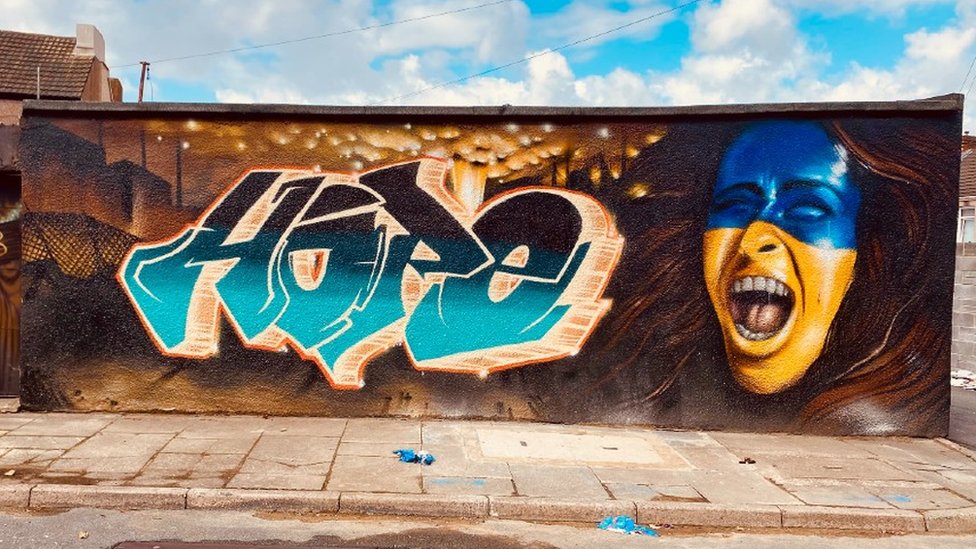The image captures an outdoor scene featuring a vibrant mural adorning a low, flat-roofed building. The graffiti art depicts a woman's face, with the top half painted in blue and the bottom half in yellow, resembling the Ukrainian flag. Her expression is intense, with her mouth open as if she is screaming, and her wavy brown hair is flowing wildly. The word "HOPE" is prominently displayed in light brown, black, and various shades of blue and white, perhaps symbolizing a rally cry of activism, particularly in support of Ukraine. In the background, there are telephone wires, a light blue sky with fluffy white and gray-accented clouds, a sand-colored building with a brown roof, and a sidewalk paved with sand-colored cobblestones, some of which are cracked. The detailed and emotive mural, with its powerful message of hope, stands out as a beacon of inspiration amidst the urban landscape.